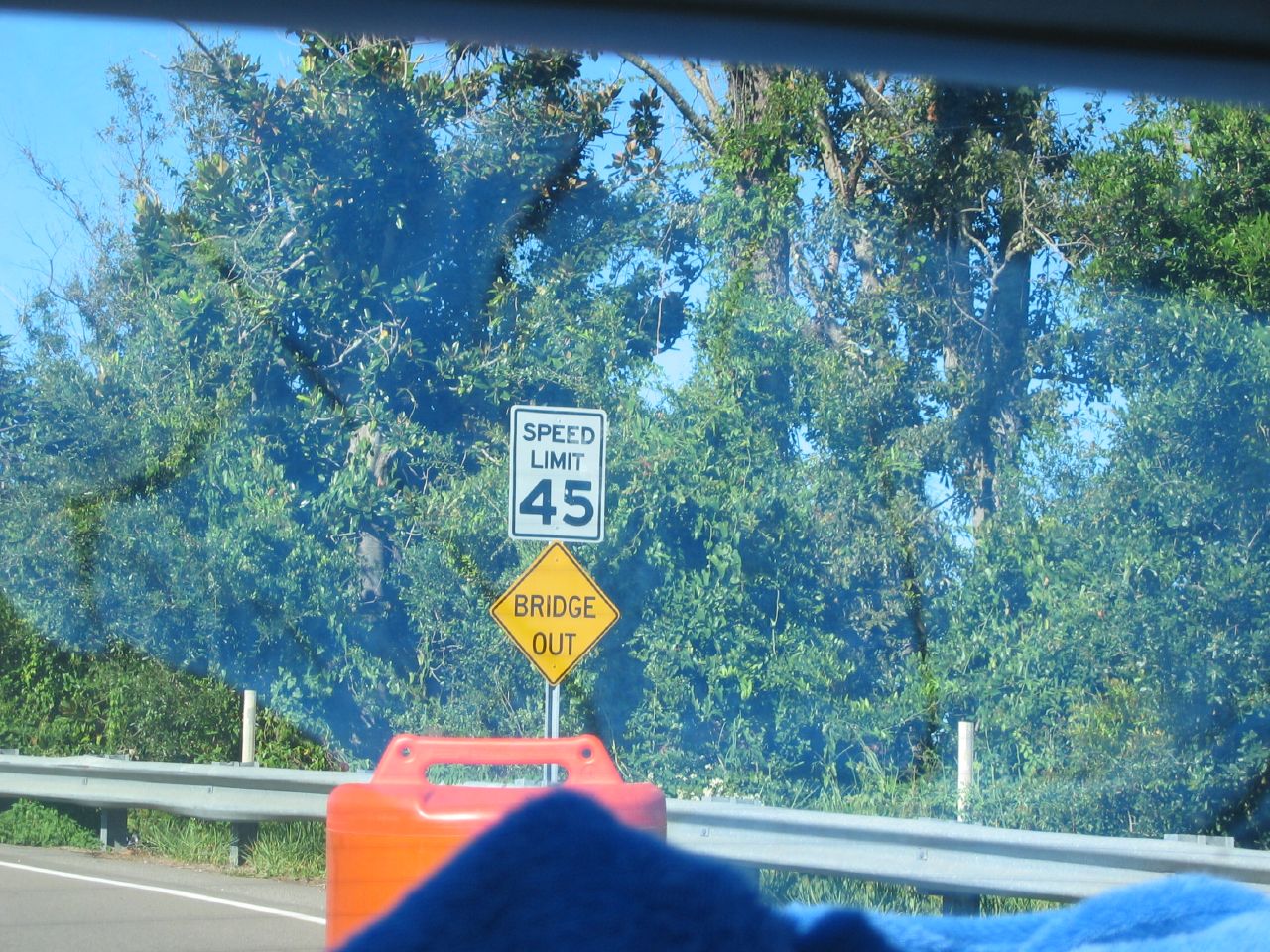A photograph taken from inside a vehicle through a slightly fogged-up window features a roadside scene. The bluish haze over the image indicates the presence of the glass through which the picture is captured. Prominently, at the center of the image, there stands a white and black speed limit sign indicating "Speed Limit 45." Directly beneath this, a diamond-shaped yellow warning sign with black letters announces "Bridge Out." To the right of these signs, a steel guardrail runs alongside a faded, gray asphalt road. Verdant green trees line the roadside, and a clear blue sky stretches out in the background.